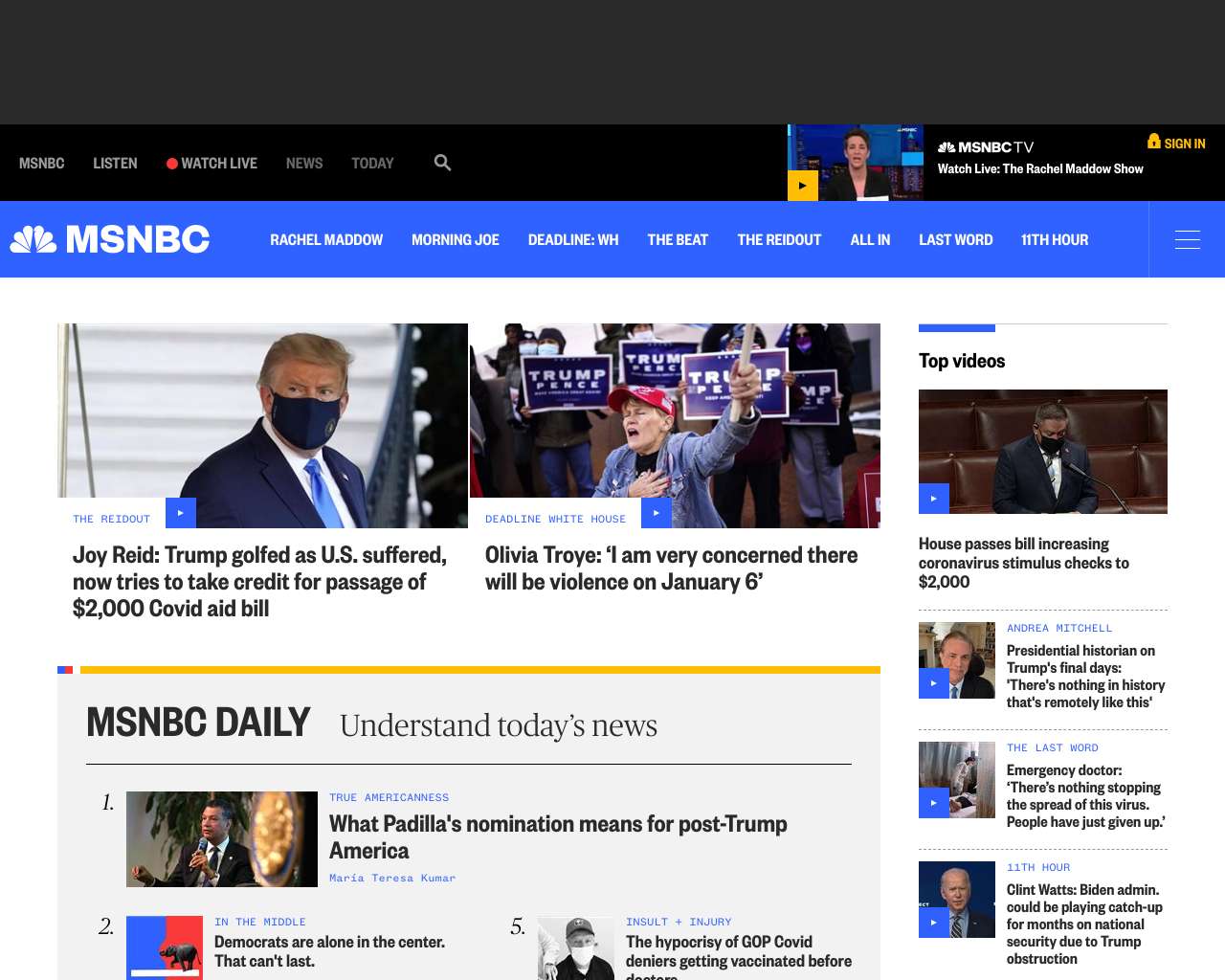**Screenshot Description: MSNBC Web Page**

This is a comprehensive screenshot of an MSNBC news web page.

**Header:**
- At the top is a black rectangular banner featuring several clickable buttons:
  - **MSNBC** (logo) 
  - **Listen**
  - **Watch Live** (highlighted by a red circle)
  - **News**
  - **Today**
  - A magnifying glass icon representing the search function
  
**Main Section:**
- On the right side, there is an image of Rachel Maddow against a blue background. She is wearing a black blazer and has short black hair.
- Next to her image, the MSNBC logo (white peacock feathers) appears along with the text:
  - **MSNBC**
  - **Watch Live**
  - **The Rachel Maddow Show** (in semi-bold white lettering)
  - **Rachel Maddow** (spelled out as R-A-C-H-E-L M-A-D-D-O-W)
- Further right, there's an orange or gold silhouette icon with the text **Sign In** underneath it.

**Subheader:**
- Below is a dark blue banner:
  - On the left, the MSNBC logo and text **MSNBC** reappear.
  - Clickable tabs labeled:
    - Rachel Maddow
    - Morning Joe
    - Deadline: White House (wh)
    - The Beat
    - The ReidOut (spelled R-E-I-D-O-U-T)
    - All In
    - Last Word
    - Eleventh Hour

**Main Content:**
1. **First News Story:**
   - Image: Donald Trump in a black tuxedo with a blue tie, white dress shirt, and black mask near white stairs.
   - Caption: **Joe Reed** - "Trump golfed as U.S. suffered new ties to take credit for passage of $2,000 COVID aid bill."
   - Second Image: An individual in a red Trump hat, jean jacket, black undershirt, with **Trump Pence** banners in the background.
   - Caption: **Deadline: White House** - **Olivia Troye** (spelled O-L-I-V-I-A-T-R-O-Y-E): "I am very concerned there will be violence on January 6th."

2. **Other News Highlights:**
   - **Padilla's Nomination:**
     - Caption: "What does P-A-D-I-L-L-A's nomination mean for post-Trump America?"
   - **House Bill:**
     - Image: Representative in a tux, white undershirt, black mask, short brown hair.
     - Caption: "House passes bill increasing coronavirus stimulus checks to $2,000."
   - **Historical Context:**
     - Caption: "Presidential Historian on Trump's final days: There's nothing in history that's remotely like this."
   - **Emergency Doctor:**
     - Caption: "There's nothing stopping the spread of the virus. People have just given up."
   - **Clint Watts:**
     - Caption: "Clint Watts (spelled C-L-I-N-T W-A-T-T-S): Von Neumann couldn't be playing catch-up for months on national security due to Trump obstruction."

This screenshot captures the rich, detailed layout of an MSNBC news web page with its navigational elements, featured news stories, and relevant imagery.